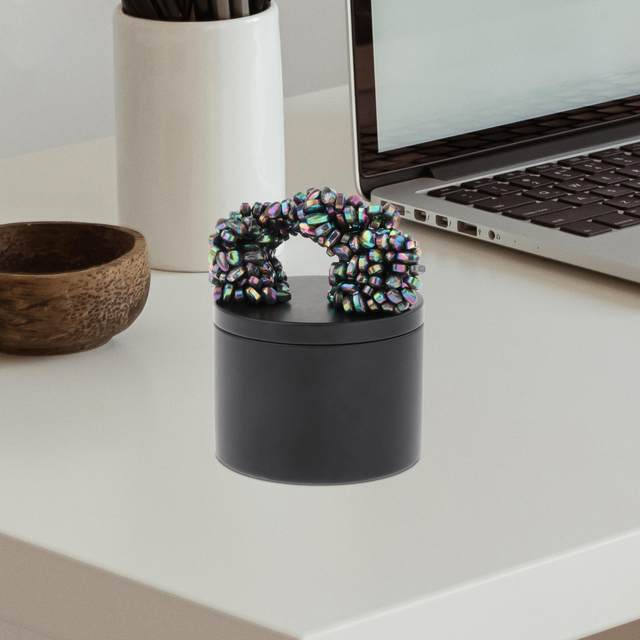This image captures a neatly arranged white desktop showcasing several distinct objects. On the right edge of the photograph, an open laptop partially appears, hinting at a working setup. Besides the laptop, a sleek white water bottle with a black rim top stands out. Adjacent to the bottle is a hand-carved wooden bowl, dark brown in color, approximately four inches in diameter and two to three inches deep, currently empty. Dominating the center of the image is a black cylinder, about three inches in both height and diameter. Atop this cylinder, an arch-shaped structure is formed from vibrant, multicolored magnetic pieces, giving the photo a playful touch. The overall setting is clear and organized, providing a harmonious blend of practical and artistic elements on a pristine white desk.